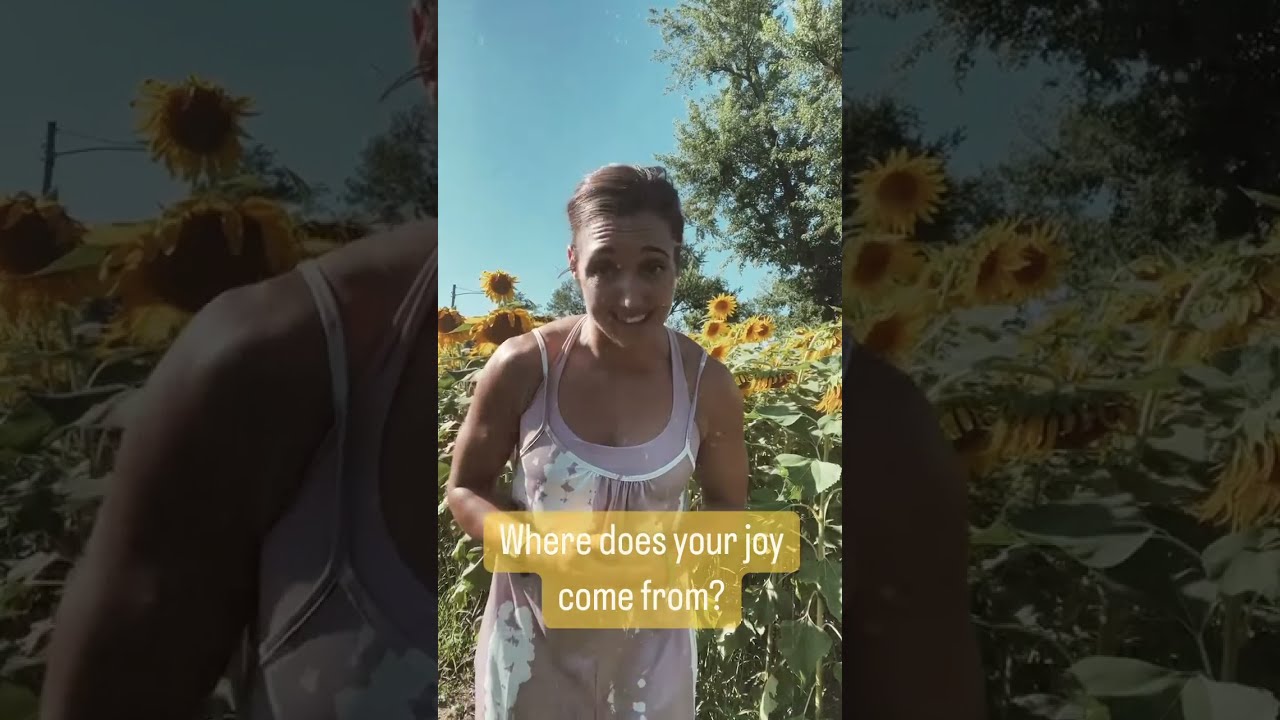A woman in her mid to late 20s stands in a vibrant field of towering sunflowers, each blossom reaching about five to six feet high. She wears a light pink sundress with thin shoulder straps over a semi-transparent, flowery overlay, and her brown hair is tied back into a neat bun, accentuating her expressive, wide-eyed smile. The image shows her from her knees up, captured in a vertical picture or video mode reminiscent of a social media post, possibly from Instagram or TikTok. She stands at the center of the frame with her elbows bent at 90 degrees in front of her waist, giving an impression of surprise and joy. Behind her, a slightly hazy, bright blue sky is visible, along with a tall oak tree and a streetlight post adding depth to the serene backdrop. Overlaying the image is a text in white font with a yellow outline that reads, "Where does your joy come from?" The image is segmented into three sections, with the middle showcasing the woman and the left and right sections being zoomed-in, half-lit parts of the central image.